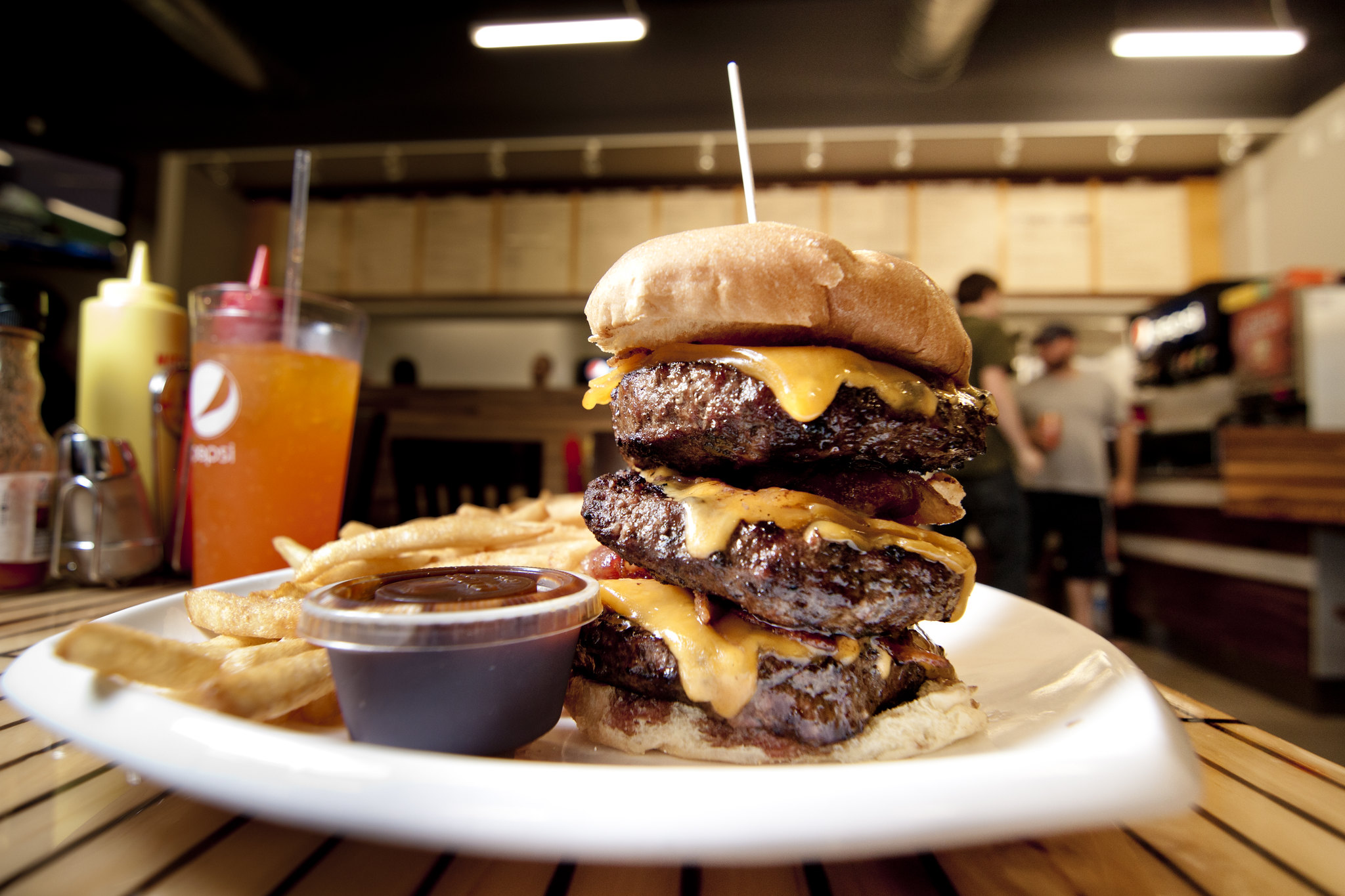The photo, taken in a restaurant, showcases a close-up of a well-composed plate of food on a white plate. In the foreground, the centerpiece is a towering triple hamburger, each of its three large beef patties adorned with a slice of cheese and possibly bacon nestled between them. The hamburger is stacked high on a bun, secured neatly with a skewer piercing through its center. Arranged around the burger are golden french fries and a small plastic container with a lid that appears to contain a brown barbecue sauce. 

To the left of the plate, a tall plastic cup branded with "Pepsi" holds an orange beverage accented with a straw. Accompanying the drink are classic condiment bottles—mustard and ketchup—and a salt and pepper shaker. The background is artistically blurred, bringing focus to the meal, yet it subtly reveals two men standing by a soda fountain, near where orders are placed in the restaurant.